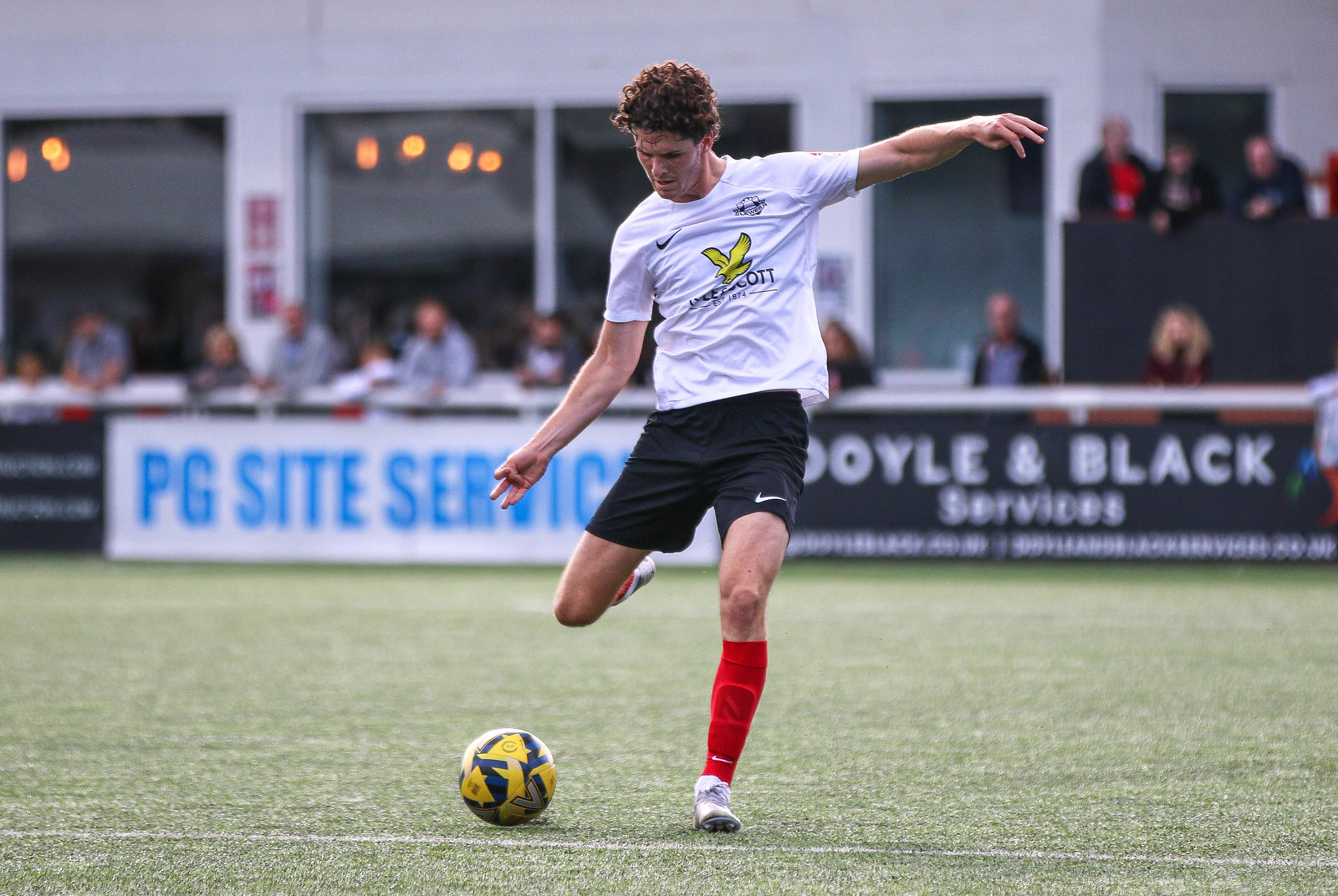This detailed color photograph captures a young soccer player poised to kick a blue and gold soccer ball on a light green artificial turf field. The player, positioned centrally in the image, is decked out in white shoes, red knee-high socks, black Nike shorts, and a short-sleeved white t-shirt adorned with a yellow bird. His reddish-brown wavy hair adds to his dynamic stance. Behind him, two tables with seated individuals, likely officials or judges, are visible, flanked by advertisement banners reading "PG Site Service" and "Doyle and Black Services." This vibrant scene is framed against the backdrop of the advertisement fencing and an audience, enhancing the energetic atmosphere of the sporting event.